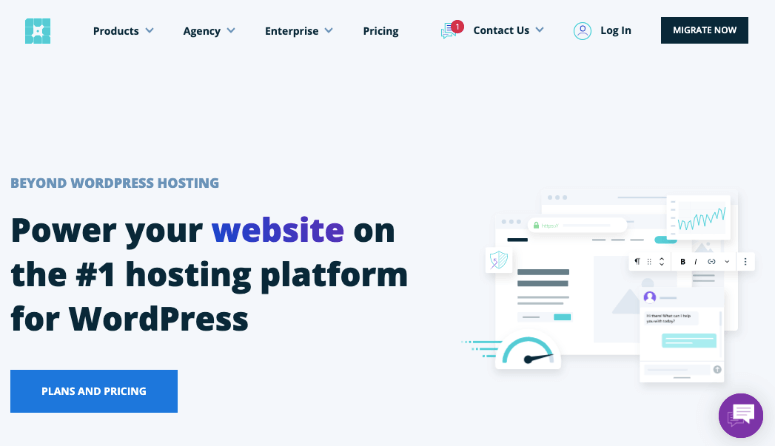A detailed and cleaned-up caption for the image:

"This image is a desktop screenshot displaying a promotional webpage for a WordPress product titled 'Beyond WordPress Hosting.' The background features an off-white hue with a hint of blue. Dominating the left side of the image is the heading 'Beyond WordPress Hosting' written in small dark blue letters. Below it, in large black text, is the statement, 'Power Your Website on the number one hosting platform for WordPress.' Directly underneath this statement, there is a prominent blue button labeled 'Plans and Pricing.'

On the right-hand side, the image showcases a simplified diagram of a blog, illustrating various features of the hosting platform. The top of the page includes a navigation bar with several dropdown options such as 'Products,' 'Agency,' 'Enterprise,' 'Pricing,' and 'Contact Us' accompanied by a text message icon. Additionally, there is a 'Login' button marked with a user profile icon and a 'Migrate Now' button, which is a dark blue rectangle with the text 'Migrate Now' in white font."